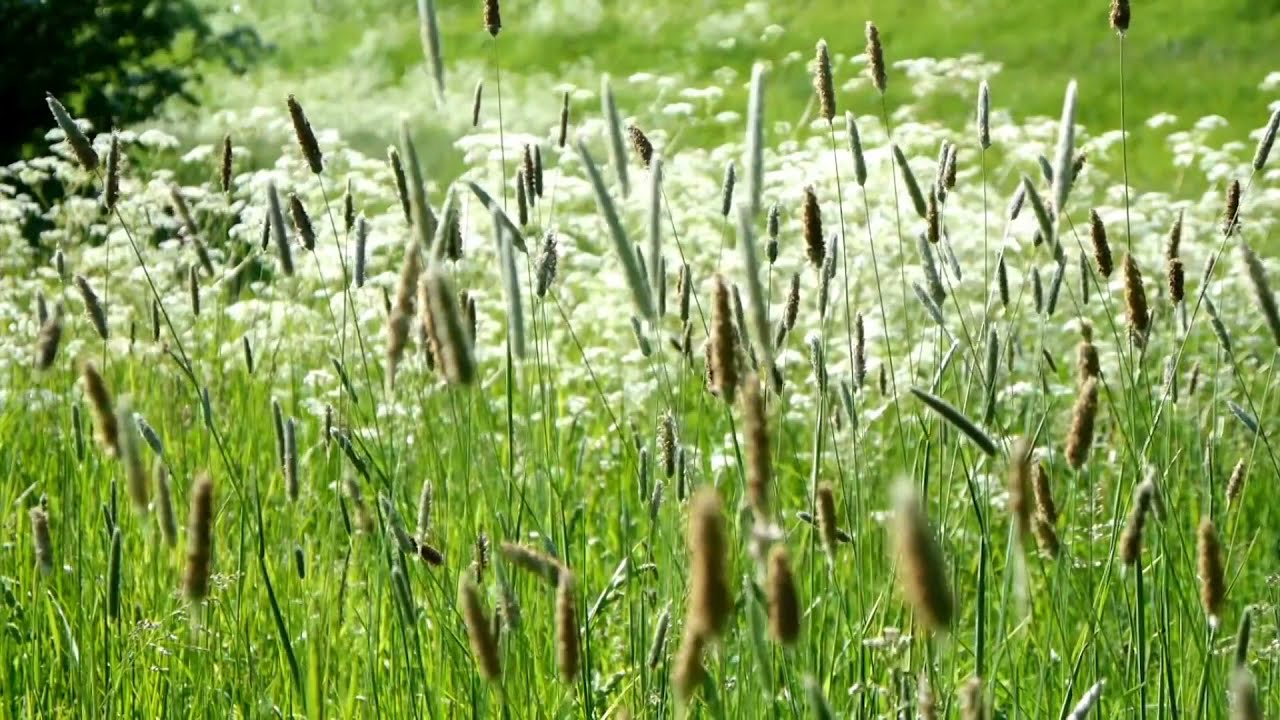The image depicts a close-up view of a lush, green countryside field brimming with tall, vibrant green grass. Interspersed among the grass are numerous cattails, characterized by their long green stems and fuzzy tops, some light brown resembling hot dogs, and others pure white. These cattails are prominently featured, standing upright and scattered throughout the scene. In the background, there's a dense array of tiny white flowers, illuminated brightly by daylight, giving a striking contrast against the green foliage. Behind this floral display, the field stretches out into a verdant, slightly hilly expanse dotted with green trees and shrubbery, adding depth and richness to the landscape. The bright light enhances the vivid colors, creating a natural and serene countryside panorama captured during the daytime.